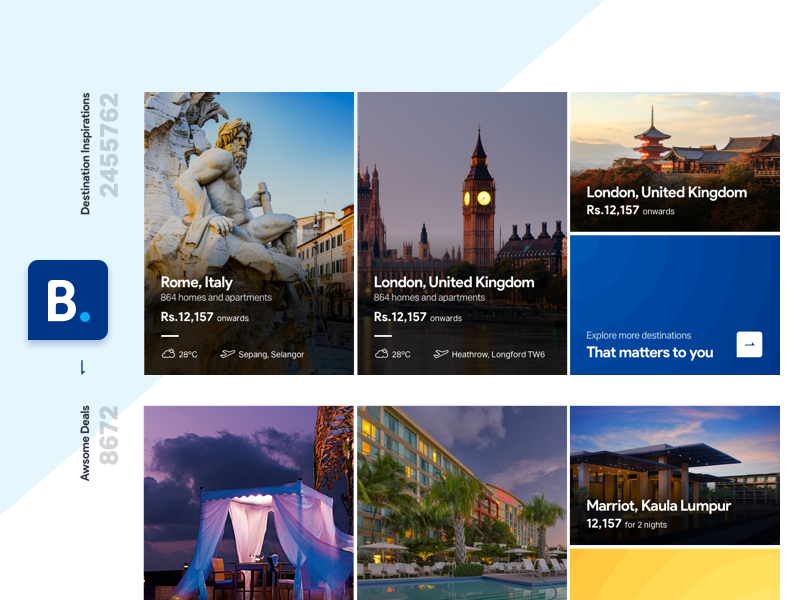On the left-hand side of the image, there is vertical text displaying "Awesome Deals: 8,672" in a small black font. At the top of this section is a white letter "B" in a blue square, which also has a small aqua blue circle at the bottom right corner. Directly above "Awesome Deals" is more vertical text that reads "Destination Inspirations." Adjacent to this is a gray number, "2,455,762." The main section of the image is composed of several blocks, each representing different travel destinations. One block features Rome, Italy, with an image of a statue. Another block showcases London, United Kingdom, followed by a block for Kuala Lumpur, Malaysia.